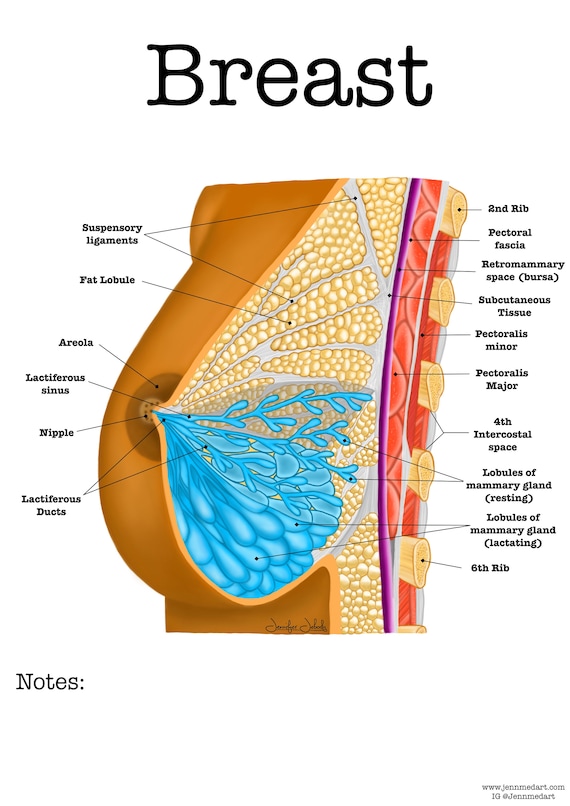This detailed anatomical diagram depicts a cross-section of a woman's breast, labeled "breast" at the top in black lettering. The image highlights various structures within and behind the breast. Inside the breast, we see suspensory ligaments, tan-colored fat lobules, and the areola, leading to the lactiferous sinus and ducts. The ducts branch out into lobules of the mammary gland, with distinct areas indicating resting and lactating states. The diagram also shows the relationship of the breast to surrounding anatomy, depicting structures such as the second and sixth ribs, pectoral fascia, retromammary space, bursa, subcutaneous tissue, and the pectoralis minor and major muscles. Detailed labeling provides clarity on the fourth intercostal space as well. A field at the bottom of the diagram is designated for notes, offering space for additional commentary or annotations.